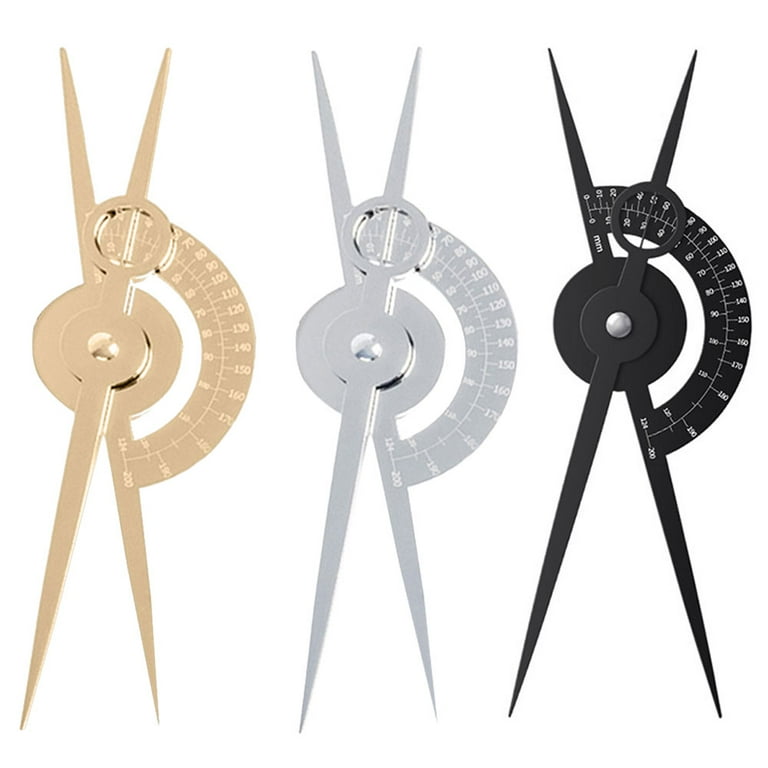This color photograph, oriented in landscape, showcases three identical geometric measuring tools that combine a protractor and a compass. These tools, typically used for mathematics, feature a central rotating dial with sharp needle points at both ends. Each instrument has a straight edge at the bottom, also ending in sharp points. Positioned from left to right, the tools are distinguished by their finishes: light brown (gold) on the left, silver in the middle, and black on the right. Notably, the black tool includes a more prominent silver bolt at the center. Numeric notations in white text are visible along the arc of each protractor. The background is a pure white, giving the impression that the instruments are floating. The photograph adheres to a style of Photographic Representationalism, Realism, and Product Photography.